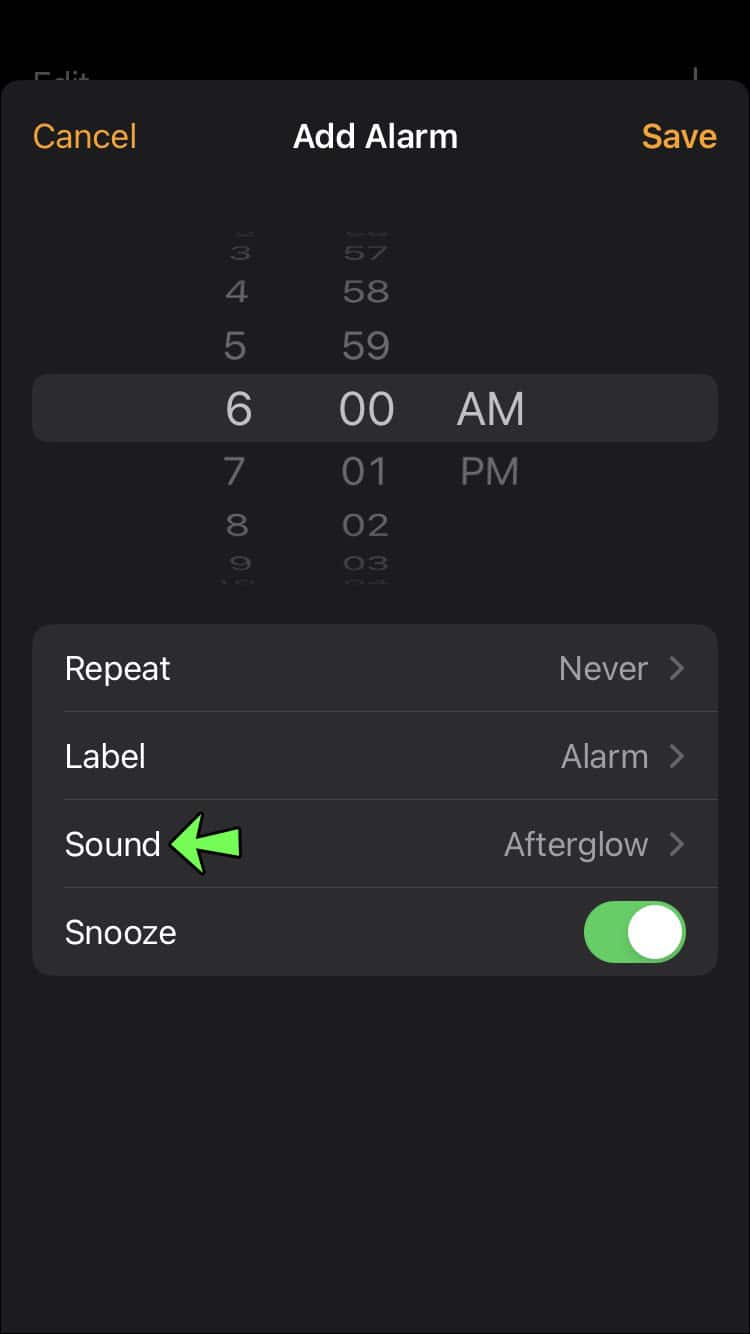Screenshot of a cell phone alarm setting screen with a black background. At the top of the screen are the options "Cancel," "Add Alarm," and "Save." Below these options, there are multiple selectable times, with 6:00 a.m. chosen as the designated alarm time. Beneath this, various settings are listed, including "Repeat: Never," "Label: Alarm," "Sound: Afterglow," with a neon green arrow pointing specifically to the "Sound" option. The "Snooze" feature is enabled, indicated by a slider button in the "on" position. The image is purely graphical with no photographic content and does not include any people, animals, plants, vehicles, or buildings.